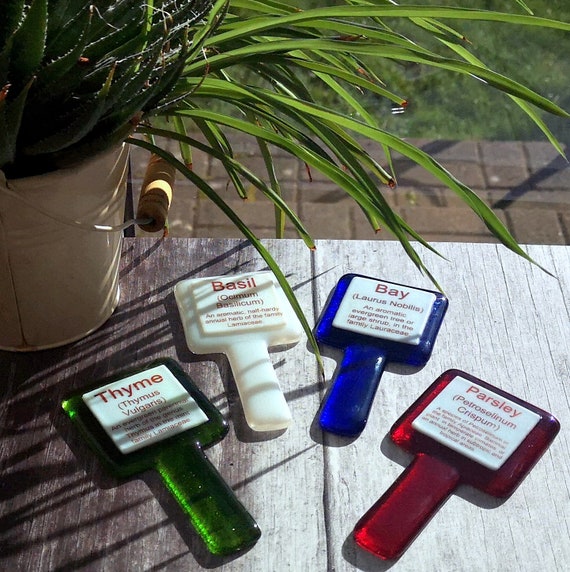The photograph reveals a beige pail with a handle housing a potted plant, likely lemongrass, featuring long, green blade-like leaves. This plant sits isolated to the left on a dark wooden table, bathed in sunlight that casts shadows onto the surface. Positioned centrally and towards the bottom of the image are four rectangular fused glass plant labels with small descriptive text underneath the names, which are difficult to read. The labels are color-coded: thyme on green, basil on white, bay on blue, and parsley on red. This arrangement is set against a background of brown paved tiles and a patch of green grass that adds an earthy vibe, suggesting a rural or suburban environment.